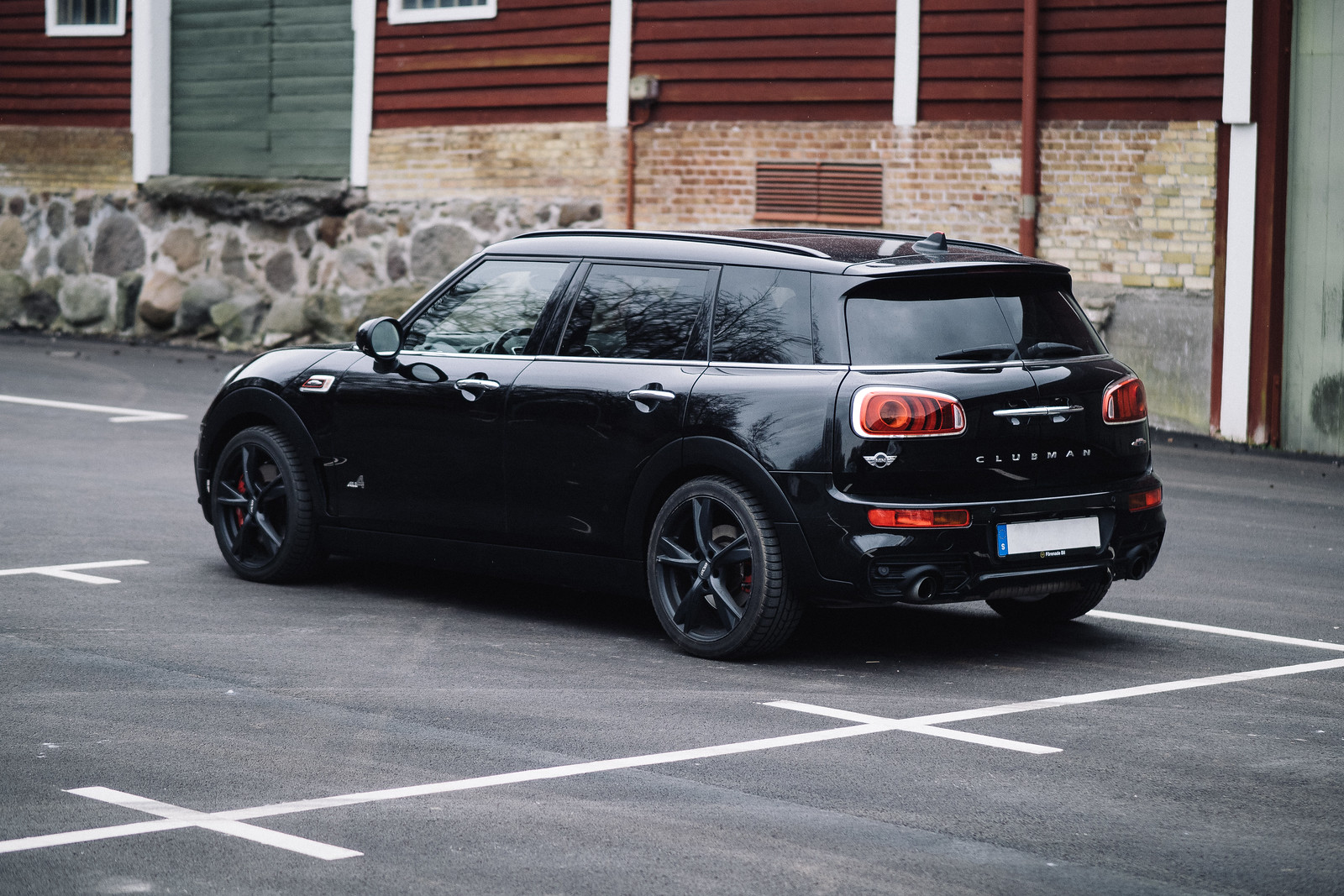A black Mini Cooper Clubman, a 4-door hatchback, is parked in a parking space marked by white lines and white crosshatches on a grayish-black asphalt lot. The car, which sits low to the ground, features roundish rectangular red taillights and silver accents on the trunk and taillights. Its back window, part of the hatch, is narrow and slightly elevated. The vehicle has black metallic rims, tinted rear windows, and a front driver's side window that is unobstructed. Additionally, there is an exhaust on the driver's side rear and a satellite radio antenna on the roof. The license plate area displays a white rectangle with a blue tab. The car is parked in front of a building with a partial stone wall that reaches a window framed in white with horizontal green shutters. Above the stone section, the building has horizontal wooden planks and white trim, with the lower portion featuring a mix of red and white bricks and a cobblestone platform.